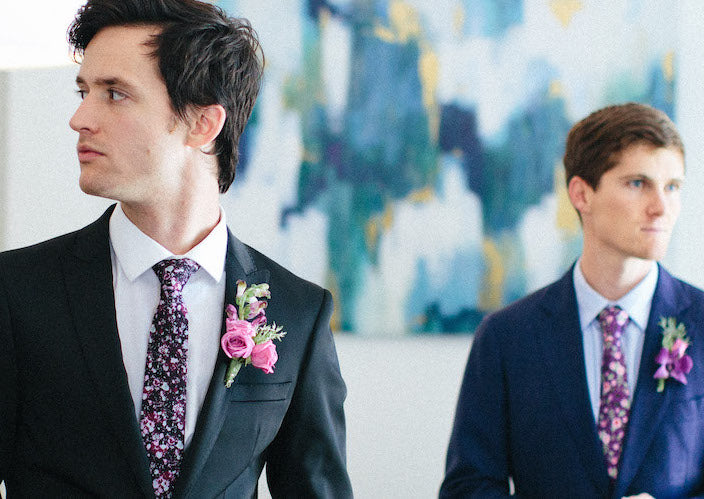The photograph features two men in suits, distinguished by their attire, floral accessories, and slightly differing appearances. The man on the left, prominently positioned in the foreground, wears a black suit paired with a white shirt and a black tie adorned with a striking pink floral pattern. His dark brown, medium-length hair is neatly combed, and he has brown eyebrows and a hint of facial hair. A pink flower boutonniere with green accents embellishes his lapel. He gazes to his right, providing a clear view of his profile. 

In the background, out of focus, stands the second man, dressed in a navy blue blazer with a light blue shirt and a complementary purple tie that also features pink flowers. His lighter brown hair is slightly shorter and styled in a more casual manner. His boutonniere, a mix of purple and pink flowers with green leaves, decorates his lapel. He looks towards the right side of the image. Both men are captured in a setting that suggests a formal event, underscored by the presence of a large, blurred artistic painting in the background. This painting is an abstract composition with a vibrant mix of blue, green, yellow, and white hues.